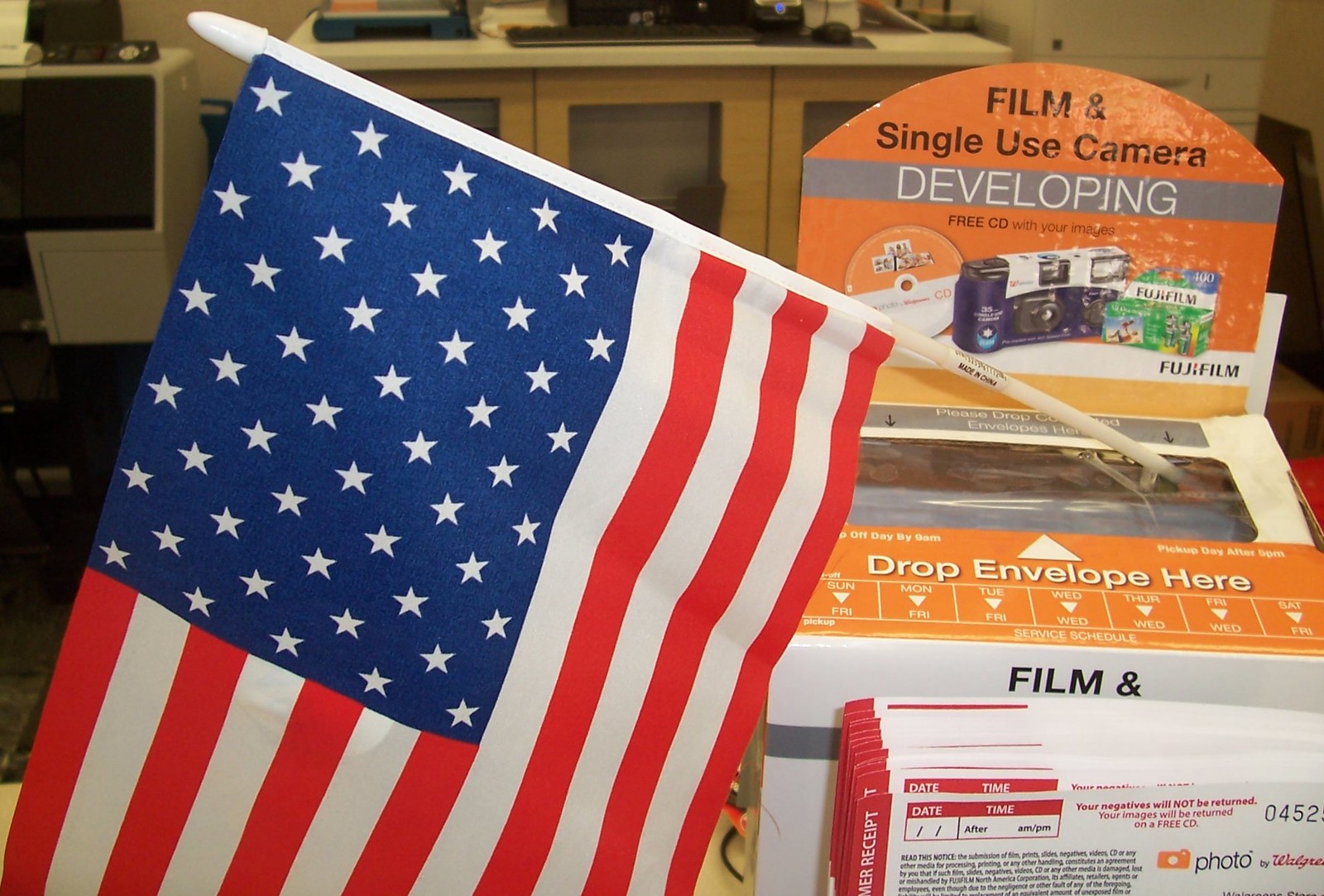The image depicts an indoor scene at a store, likely a photo or photocopy store, featuring a dedicated setup for film and single-use camera development. The focal point is a drop box located on the right side, adorned with various elements. The box displays prominent white text against a gray background, stating "Film and Single-Use Camera Developing." Below this text, there are pictures of disposable cameras and film, specifically noting Fujifilm. The box features an area in the lower right corner with several envelopes for customers to use, where they can fill in details such as the date, time, name, and contact number before dropping them in for processing.

An eye-catching feature is a plastic pole with an American flag sticking out of the box, its blue field and red and white stripes prominently visible on the left side of the image. The envelope drop-off slot itself is marked with "Drop Envelope Here" in white letters. The scene is set against an orange background, with additional colors including red, white, blue, black, gray, and a handful of other hues like purple, green, yellow, and tan. In the background, there are indistinct counters and cabinets, hinting that this might be part of a larger workstation or service counter. The absence of people and the general arrangement suggest a functional, yet somewhat dated, store interior focused on photographic services.